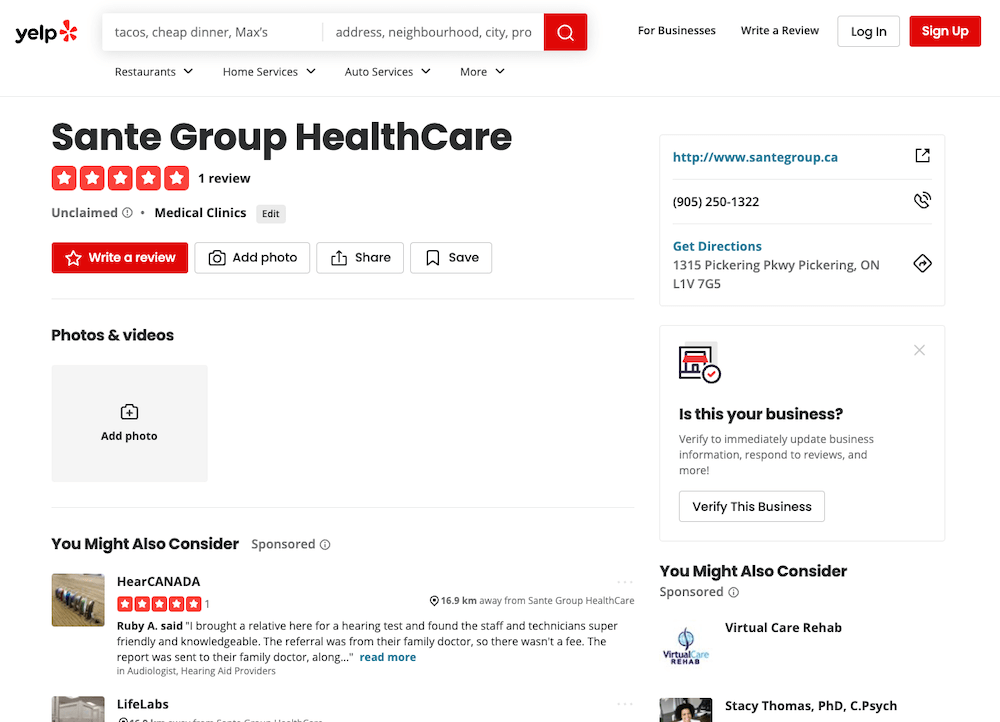The image showcases the result of a Yelp search, prominently featuring the familiar Yelp search bar at the top alongside the Yelp logo, characterized by black text and a red floral emblem. The primary search result highlighted in the image pertains to "Sante Group Healthcare," a healthcare provider that has garnered one review, rated at five stars, for its medical clinic services. 

Beneath this review, there are prompts allowing users to write their own review and add a photo or video. Additionally, the image includes a section with alternative search suggestions; the first recommended option is "Here Canada," which also boasts a solitary five-star review.

On the left-hand side of the page, users can find a link to Sante Group Healthcare's website, along with their contact phone number, and an option to get directions to the clinic. There's also a feature for business verification and further recommendations of related searches. All text is displayed in black and red against a clean white background, maintaining a consistent and visually organized layout.